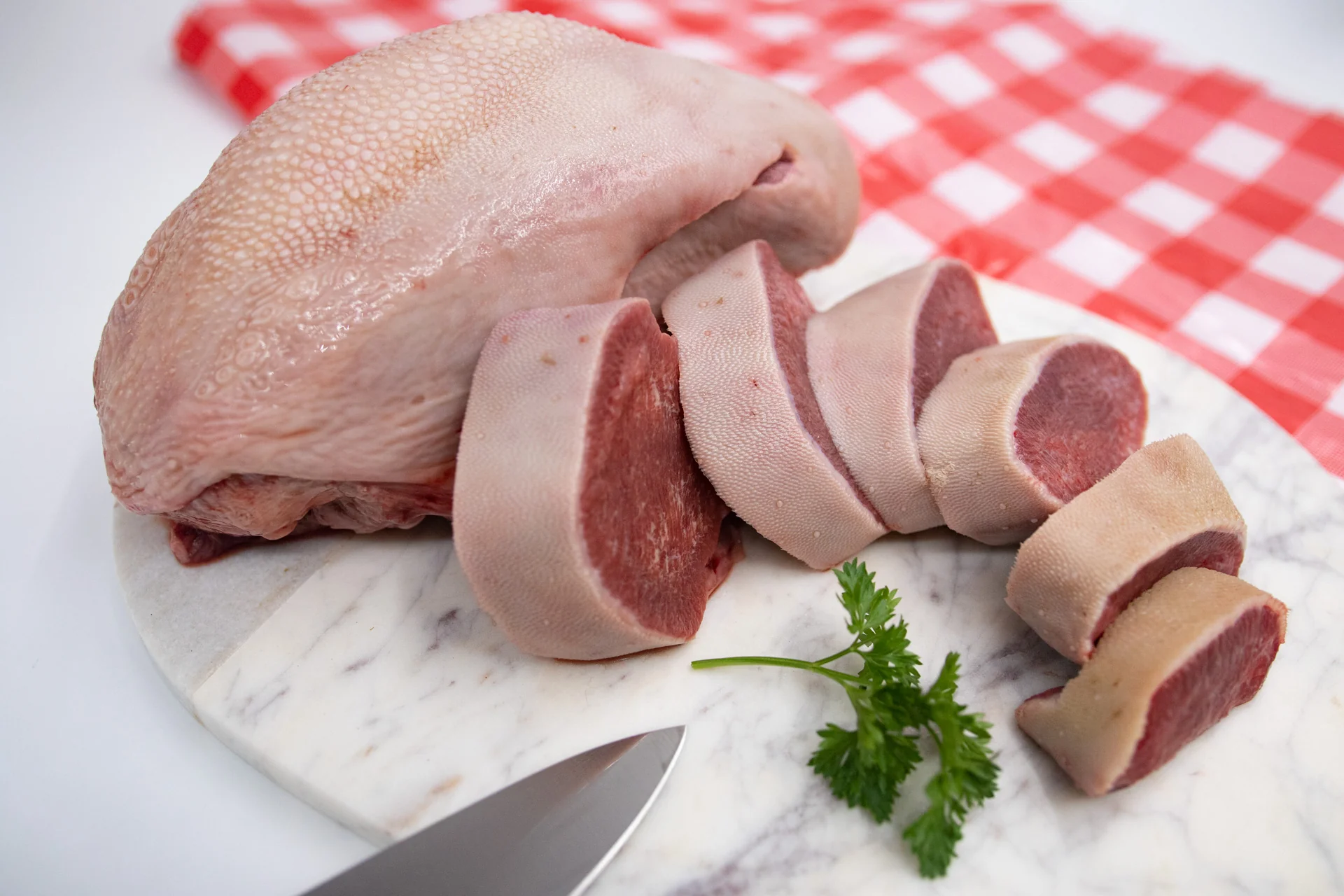The image depicts a slab of raw meat with a pink exterior and a red interior, which appears to be beef, not chicken. The main piece of meat sits on a gray and white marble cutting board, accompanied by six neatly sliced pieces in front of it. On the cutting board, a sprig of parsley is placed right in front of the meat slices, and a sharp knife is positioned at the edge, pointing towards the meat. The background features a red and white checkered cloth, resembling a picnic napkin or tablecloth, all set against a clean white backdrop. This detailed and well-composed image gives the impression of a high-quality presentation suitable for a recipe site or an advertisement.